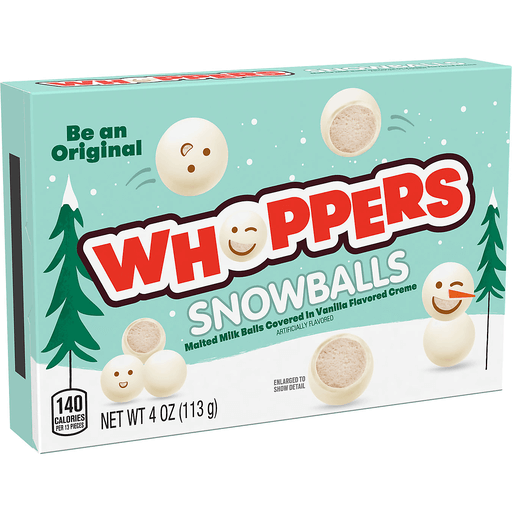This photograph showcases a special Christmas edition of Whopper's Snowballs candy, presented in a movie theater-sized box with a minty teal background. The prominent red and white Whoppers logo, outlined in black, features a festive twist where the "O" is replaced with a winking snowman's face. To the left, a skinny snow-topped Christmas tree adds a whimsical touch, while snowflakes gently fall against the backdrop. Below the logo, the text reads, "Snowballs, malted milk balls covered in vanilla flavored cream." Adding to the festive charm, two Whoppers coated in vanilla cream are depicted flying through the air like snowballs, with one cut open to reveal the malt inside. At the bottom left, nutritional information is displayed, stating 140 calories per 13 pieces, alongside a net weight of 4 ounces (113 grams). On the right, a snowman assembled from three Whoppers snowballs stands next to another simply drawn tree, reinforcing the holiday spirit. The top left corner features the phrase "Be an Original" in green, tying together this festive and detailed presentation.